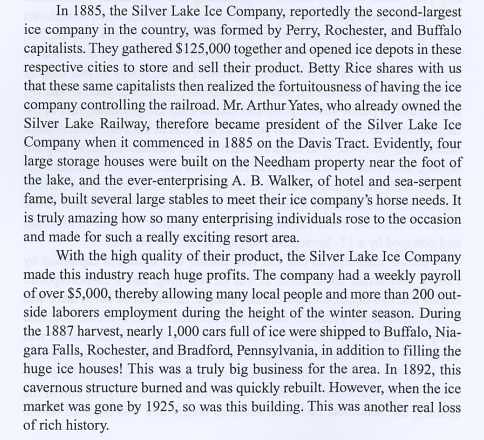The image appears to be a photograph of an old newspaper clipping featuring an article written in black Times New Roman font on an off-white or gray background. The article, titled "In 1885," recounts the formation of the Silver Lake Ice Company, reportedly the second largest ice company in the country. Founded by Perry, Rochester, and Buffalo capitalists who amassed $125,000, the company established ice depots in these cities to store and sell their product. Betty Rice notes that the founders realized the advantage of controlling the railroad, leading Mr. Arthur Yates, who owned the Silver Lake Railway, to become the company's president when it commenced on the Davis Tract in 1885. Four large storage houses were constructed on the Needham property on the lake's edge, and A.B. Walker of Hotel and Sea Serpent fame built stables to meet the company's horse needs, contributing to the area's excitement as a resort. The high-quality ice brought immense profits, with the company employing over 200 local and external laborers, boasting a weekly payroll of over $5,000. In the 1887 harvest, nearly 1,000 carloads of ice were shipped to cities like Buffalo, Niagara Falls, Rochester, and Bradford, Pennsylvania, enhancing the area's economic landscape. Unfortunately, the original structure burned down in 1892 but was swiftly rebuilt. The ice market's decline by 1925 led to the building's abandonment, marking a significant loss in the region's rich history.